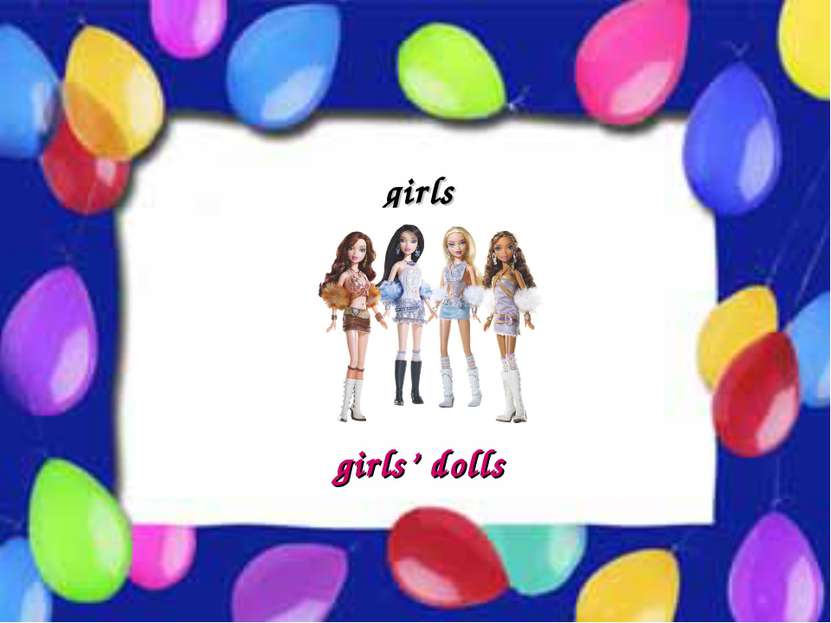This horizontal rectangular advertisement image is vividly designed with a dark blue background featuring colorful balloons scattered around, evoking a festive atmosphere. At the center sits a large white rectangle displaying four animated depictions of young girls or dolls dressed stylishly for a party. Each figure is adorned in short skirts and knee-high boots, complete with long hair in varying shades of brown, blonde, black, and red, each holding a handbag or purse. The top of the white rectangle prominently showcases the word “girls” in dark lowercase letters, and below, in bold red letters, it reads “girls dolls.” The image gives the impression of either dolls that resemble young girls or vice versa, aimed at a younger audience, possibly for a celebratory event or a product advertisement.